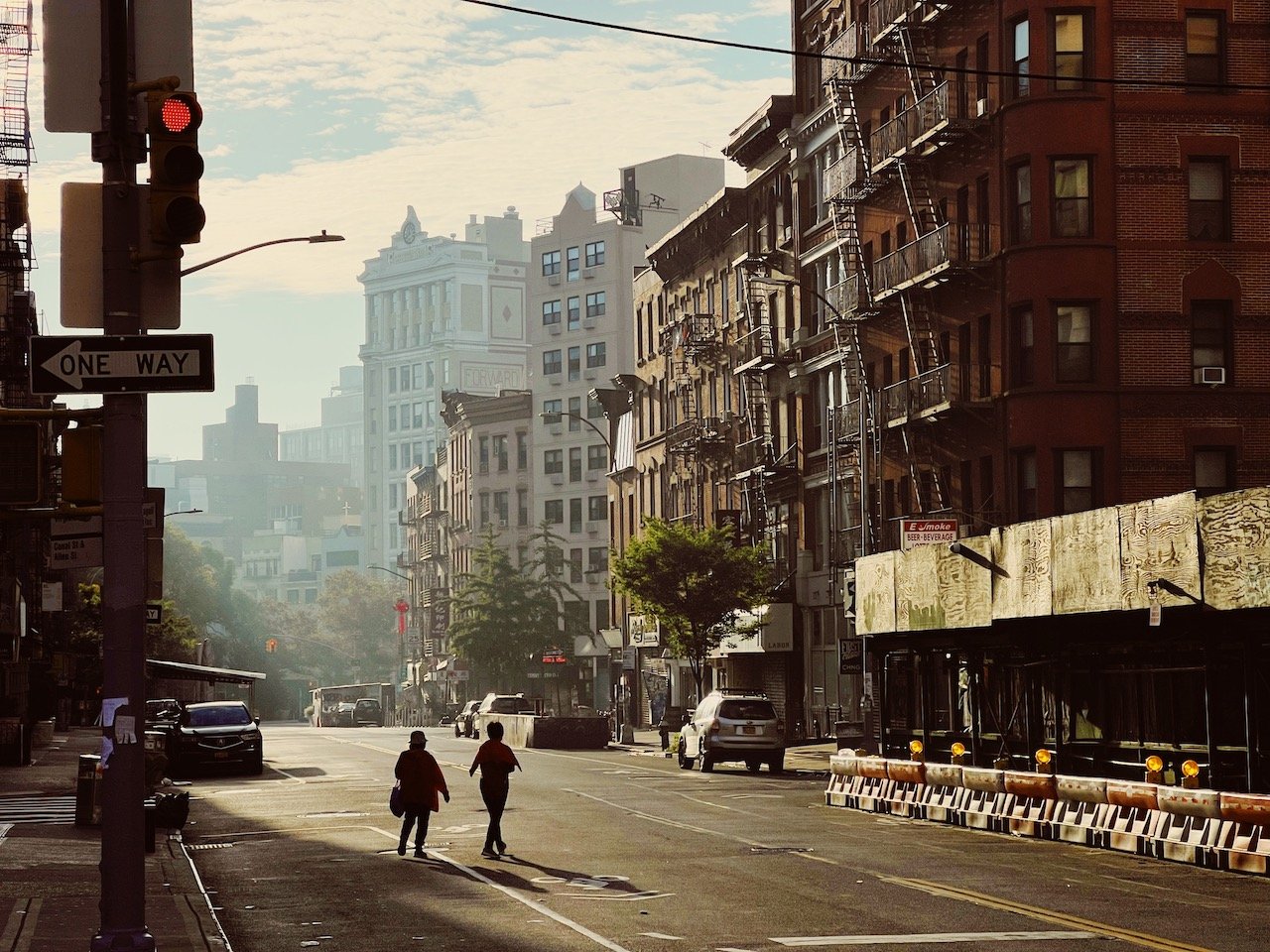The image depicts a cityscape scene filled with detail and character. Center stage are two women crossing a street diagonally, their figures silhouetted and shadowed, suggesting it might be evening or a foggy day. Surrounding them are tall apartment buildings, each adorned with metal fire escapes that snake down from one floor to the next, providing a visual testimony to the building's age, likely from the early 1900s. Some buildings even have window air conditioning units jutting out, enhancing the urban feel.

On the left side, there are noticeable road signs, including a red traffic light, a walking light, and a one-way traffic arrow, contributing to the city's bustling yet organized traffic system. Next to one apartment building, construction is underway, evidenced by big plywood boards and concrete barriers protecting the site.

The background features more tall buildings shrouded in what appears to be smog or fog, giving the scene a muted, atmospheric quality. The sky is partly to mostly cloudy, adding to the overall moody ambiance. Sparse trees punctuate the setting, but the primary focus remains on the urban landscape. Cars are parked along both sides of the street, though no vehicles are actively driving through, creating a sense of stillness amidst the inherent city movement. A notably taller and whiter building stands proudly in the background, distinct from its neighbors, and adding an element of architectural diversity to the scene.